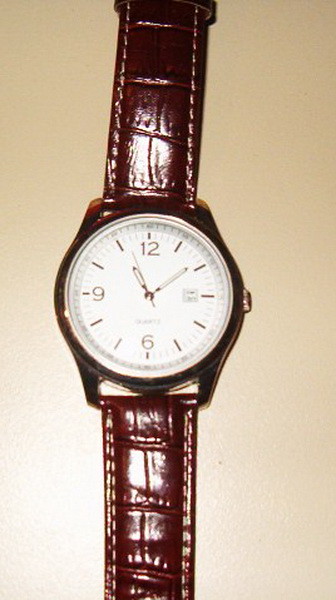The image depicts a man's wristwatch against a gradient tan background that transitions from darker at the top to lighter at the bottom. The watch features a somewhat wrinkled and crinkly leather band, colored in a reddish-brown burgundy hue with lighter tones between the lines, enhanced further by white stitching. Light reflects softly off the band, adding a subtle shine. The circular watch face is white, encased in gold trim, featuring a tiny winding knob on the side. The hour markers include prominent gold-colored digits at the 12, 9, and 6 positions. Instead of the number 3, there is a small square display showing the date. Other hour markers are denoted by angled diagonal lines. Above the number six, the word "Quartz" is inscribed, and the watch displays the time as 11:08.